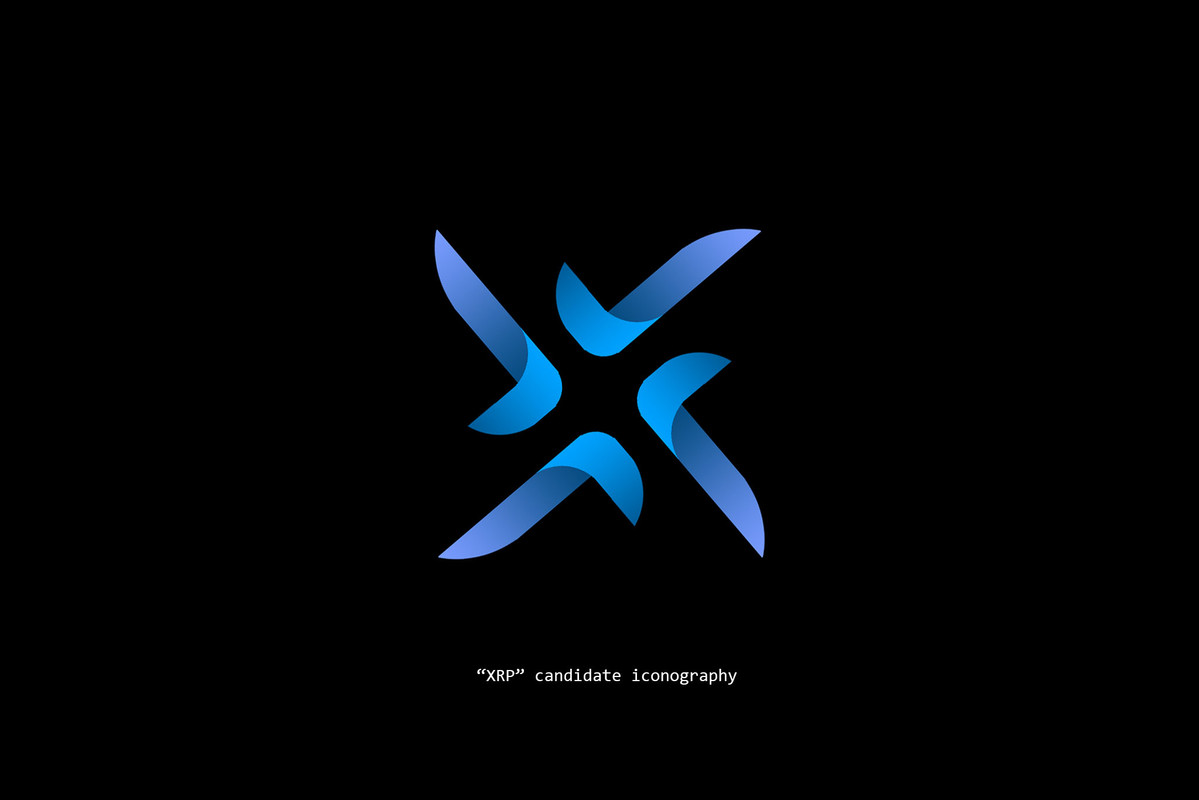This image resembles a minimalist desktop wallpaper or poster. It is designed in a flag-like, long rectangular format with a solid black background. The focal point is a centrally placed logo, which appears blue and resembles a pinwheel or windmill in shape. The logo is composed of a blue shape resembling either a backward 'L' or a capital 'J' with less curvature on the lower part. This shape is repeated four times, arranged to form an off-center 'X' pattern, reminiscent of a four-blade fan. Below the logo, in small white text, is the phrase "XRP Candidate Iconography" within quotation marks.